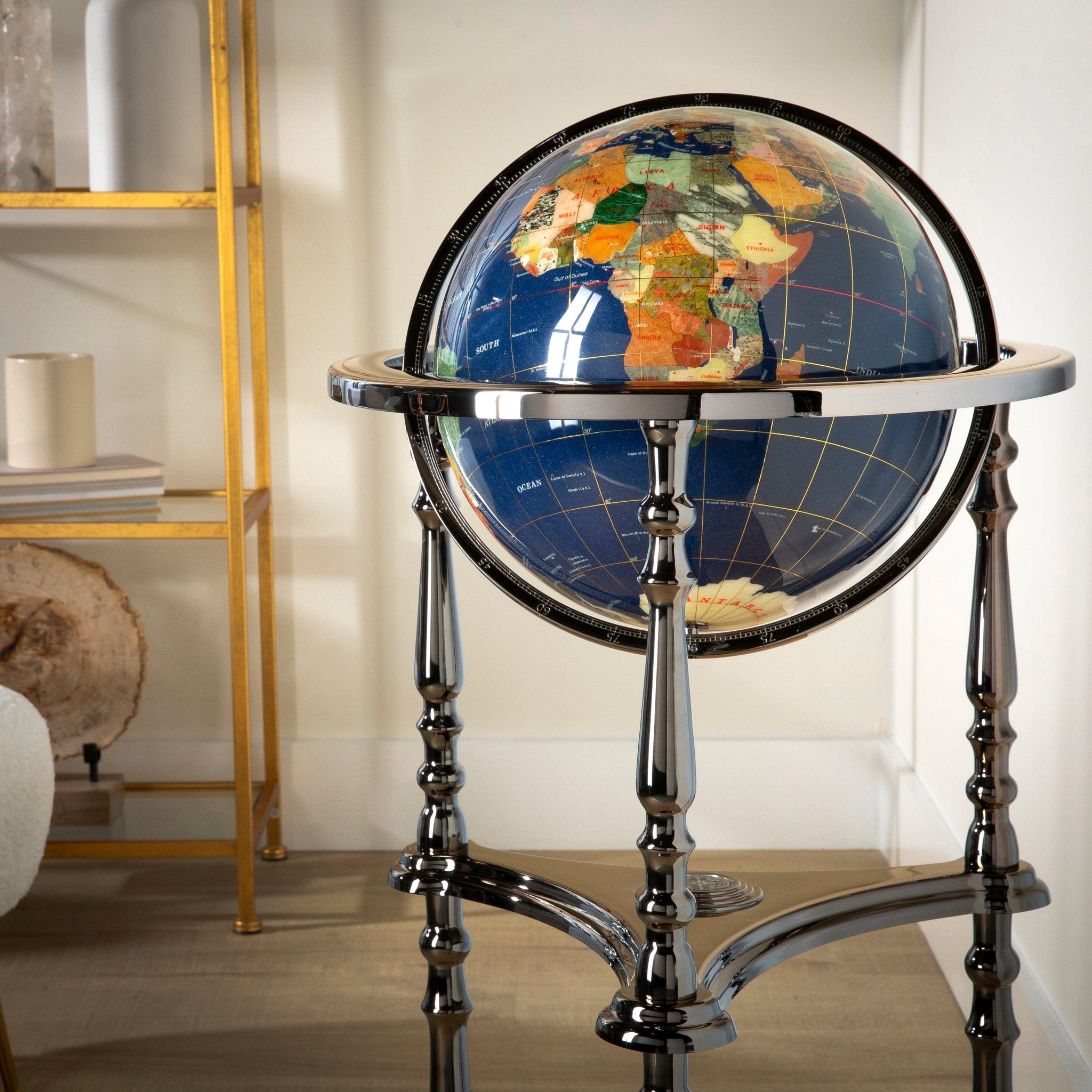The image depicts a detailed and colorful globe mounted on a glossy, dark blue tripod stand with three legs. The globe is suspended within a ring that allows it to be turned in different directions, revealing vibrant countries in Africa, colored in oranges, greens, grays, whites, and yellows, with the equator and other latitude and longitude lines clearly visible. The scene shows part of Sri Lanka and India as well. The tripod’s legs are straight and meet at the bottom to keep the stable structure, positioned on a dark brown hardwood floor. 

The room's walls are light-colored, possibly white or ivory, with thick white baseboards. To the left of the globe is a wooden étagère with glass shelves displaying various objects. The shelves hold an assortment of items, including what appears to be a cream-colored vase on the second shelf, a tall white cylindrical vase on the top shelf, and items such as a gemstone or agate stone, a candle, and books. The room, with its wooden floor and organized décor, provides a warm and sophisticated backdrop to the dynamic centerpiece of the globe.